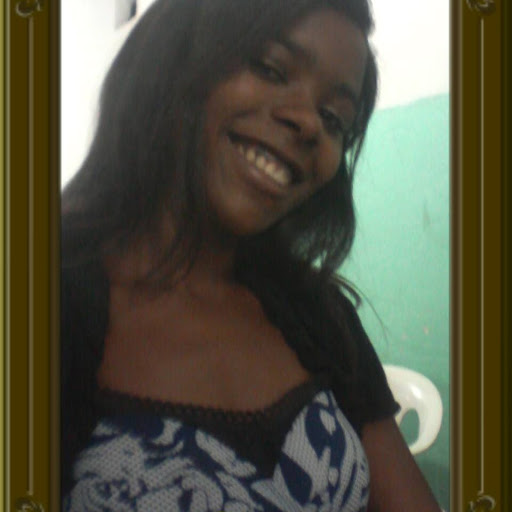The image captures a young, dark-complexioned woman standing within a textured brown door frame. She appears to be either African American or Middle Eastern with medium-length black hair and minimal makeup. Her head is tilted gently to the side, and she smiles warmly, displaying her teeth and upper gums. She is dressed in a black vest that covers her shoulders and upper arms, worn over a floral-patterned blouse featuring shades of white, dark blue, and purple. Additionally, a black lace garment is partially visible beneath her blouse. The woman stands slightly leaning against the doorway, which centers her directly in the photo. Behind her, a white plastic chair is positioned against a wall that transitions from green at the bottom to white towards the top. No text is present in the image, and the overall color palette includes brown, black, white, purple, teal blue, and green. The setting suggested by the surroundings may indicate that the photo was taken in a third-world country.